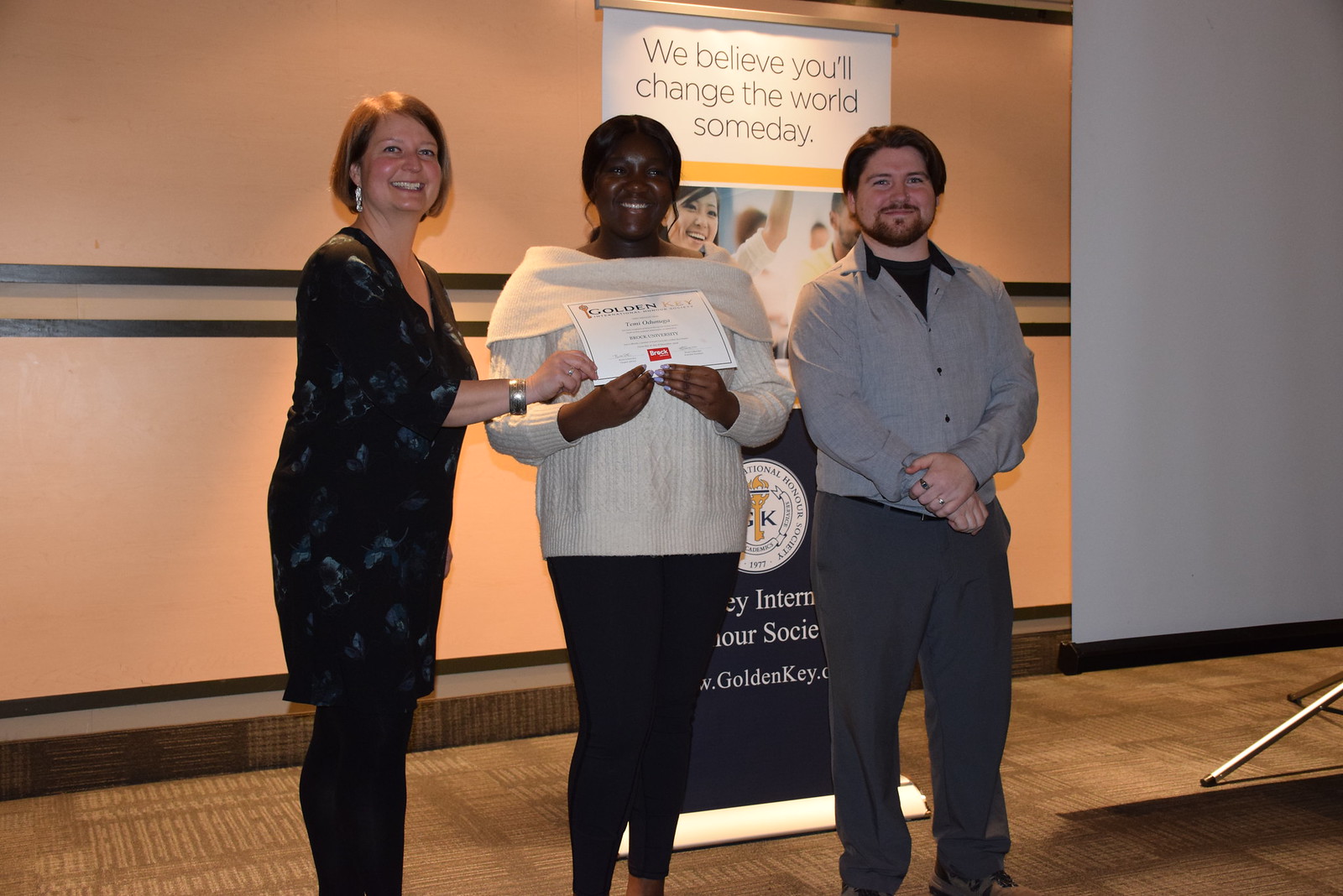The rectangular indoor photograph captures a serene moment during what appears to be an award ceremony or seminar set in a conference room. Dominating the background is a partially visible banner that reads, "We believe you'll change the world someday," accompanied by a photograph of a woman and the partially obscured text mentioning an honor society and a website. To the right of the banner stands a blank projection screen.

In the foreground, three people smile warmly at the camera. On the left, a woman with chin-length reddish-brown hair wears a black dress and black tights. She is handing a certificate to a woman standing in the center, who sports a white, off-the-shoulder sweater and black leggings. Flanking them on the right is a man with dark hair, a beard, and mustache, dressed in gray pants and a gray shirt over a black t-shirt. The beige wall behind them features black stripes, adding a touch of decorum to the setting. Overall, the scene radiates a formal yet celebratory atmosphere, underscoring the sense of achievement and camaraderie.